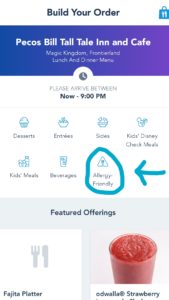**Caption:**

Despite the slight blur of the screenshot, several key elements are still visible. At the very top, in dark blue font, it reads "Build Your Order." To the right of the title, there is a shopping bag icon in blue, displaying the number 11. Just below, a purple-to-blue ombre banner prominently states "Pico's Bill Tall Tale Inn and Cafe." The text below this banner is unreadable due to the blur, but a clock icon is visible in the center with the accompanying text, "Please arrive in time," followed by "NOW - 9 PM" in grey, all caps letters. 

Below this section, there is a row of icons and text categories, although some words are indistinct. They likely represent menu categories such as "Desserts," "Entrées," "Sides," "Kids," "Delivery," "Check Meals," "Cash Meals," "Fish Meals," and "Beverages." Additionally, a section for "Allergy Friendly" items is circled in blue, suggesting it was highlighted manually, possibly for emphasis. 

The next section is titled "Featured Offerings." On the left, an icon of a fork and knife with a sheet of platter below it is present. To the right of this, there appears to be a drink icon. Below this icon, it reads "Edwalla Strawberry," depicting what seems to be a strawberry slush drink.